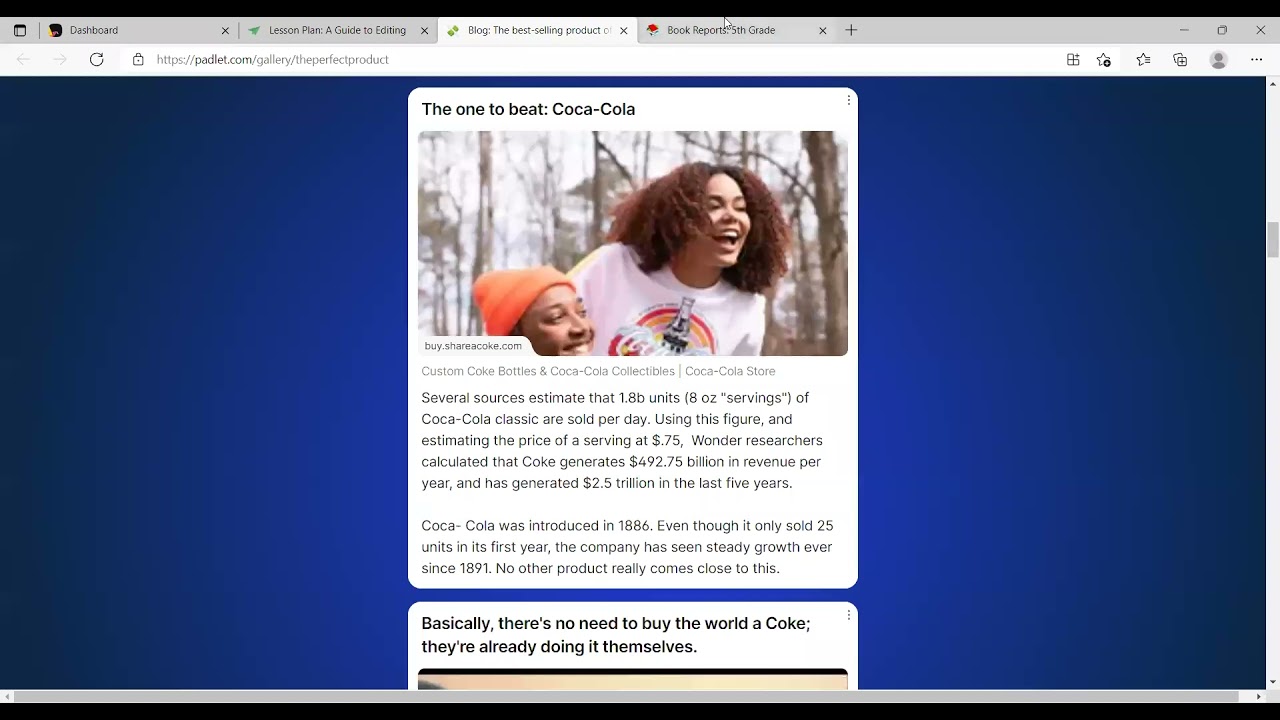**Caption:**

Under the category "Coca-Cola," the image showcases a dynamic interface with multiple tabs open at the top, including "Dashboard," "Lesson Plan: A Guide to Editing," "Blog: The Best Selling Product," and "Book Reports: Fifth Grade." Below these tabs is a search bar reading "Padlet.com, Gallery the Perfect Product."

The central focus of the image features a vibrant blue background with bold text proclaiming "The One to Beat. Coca-Cola." In the foreground, an African American woman wearing a shirt emblazoned with the Coca-Cola logo stands next to another African American individual dressed in a knit cap, whose gender is ambiguous from the image. 

Beneath this, there is a promotional note directing viewers to "buyshareacoke.com" for custom Coke bottles and Coca-Cola collectibles, and a comprehensive Coca-Cola store.

The caption continues with an interesting fact: "Several sources estimate that 1.8 billion units of 8-ounce servings of Coca-Cola Classic are sold per day. Using the price estimate of 75 cents per serving, a researcher calculated that Coke generates approximately $492.75 billion in annual revenue and has accrued about $2.5 trillion in revenue over the past five years. Coca-Cola was first introduced in 1886."